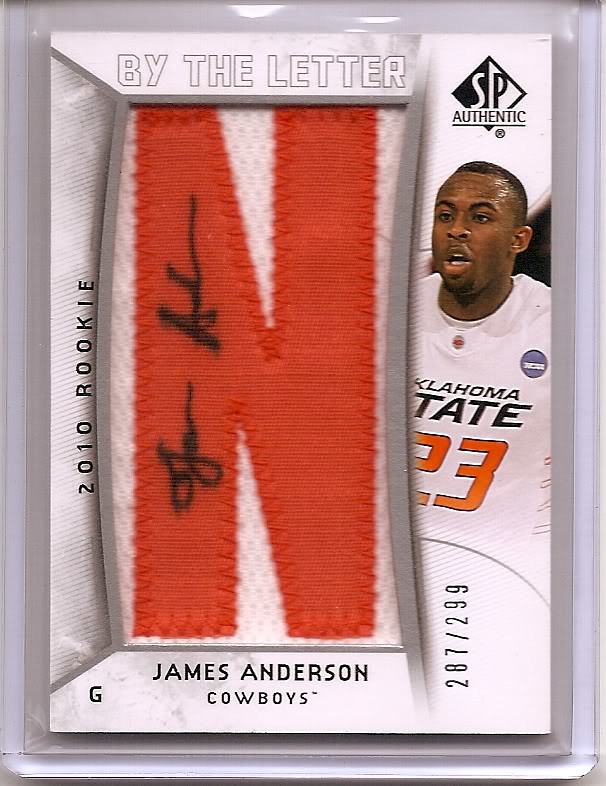The image features a meticulously presented sports memorabilia card from SP Authentic, highlighting 2010 rookie James Anderson of the Cowboys, presumably from Oklahoma State. Dominating the center of the card is a plastic window showcasing a large, orange letter "N" stitched into white fabric, which may be part of his jersey or uniform and is autographed by Anderson across the left section of the 'N.' On the right side of the card is a photograph of James Anderson wearing his number 23 jersey. Below his image, the text "287/299" suggests this is a limited edition item. Additional details include "2010 Rookie" prominently displayed and a small black letter "G" in the bottom left corner, possibly indicating his position as a guard. The entire card appears to be laying in a bin or container when the photo was taken.